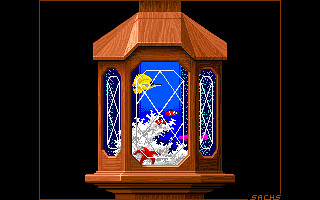The image depicts a uniquely styled 2D fish tank with a design reminiscent of an antique street lamp. The structure, shaped like an octagon or hexagon, is framed in wood with transparent glass panels. Inside, the glass encloses a scene filled with a vibrant blue background, mimicking water. At the center of the tank lies a white coral formation, resembling a small, spiky bush. Resting lifelessly on the coral is a red starfish, its limbs slack and drooping as though melted onto the coral. Accompanying this melancholy scene are a few lively orange fish and a single yellow fish, swimming within the blue depths. In the bottom right corner of the scene is the word "sack," adding a mysterious touch to the composition.